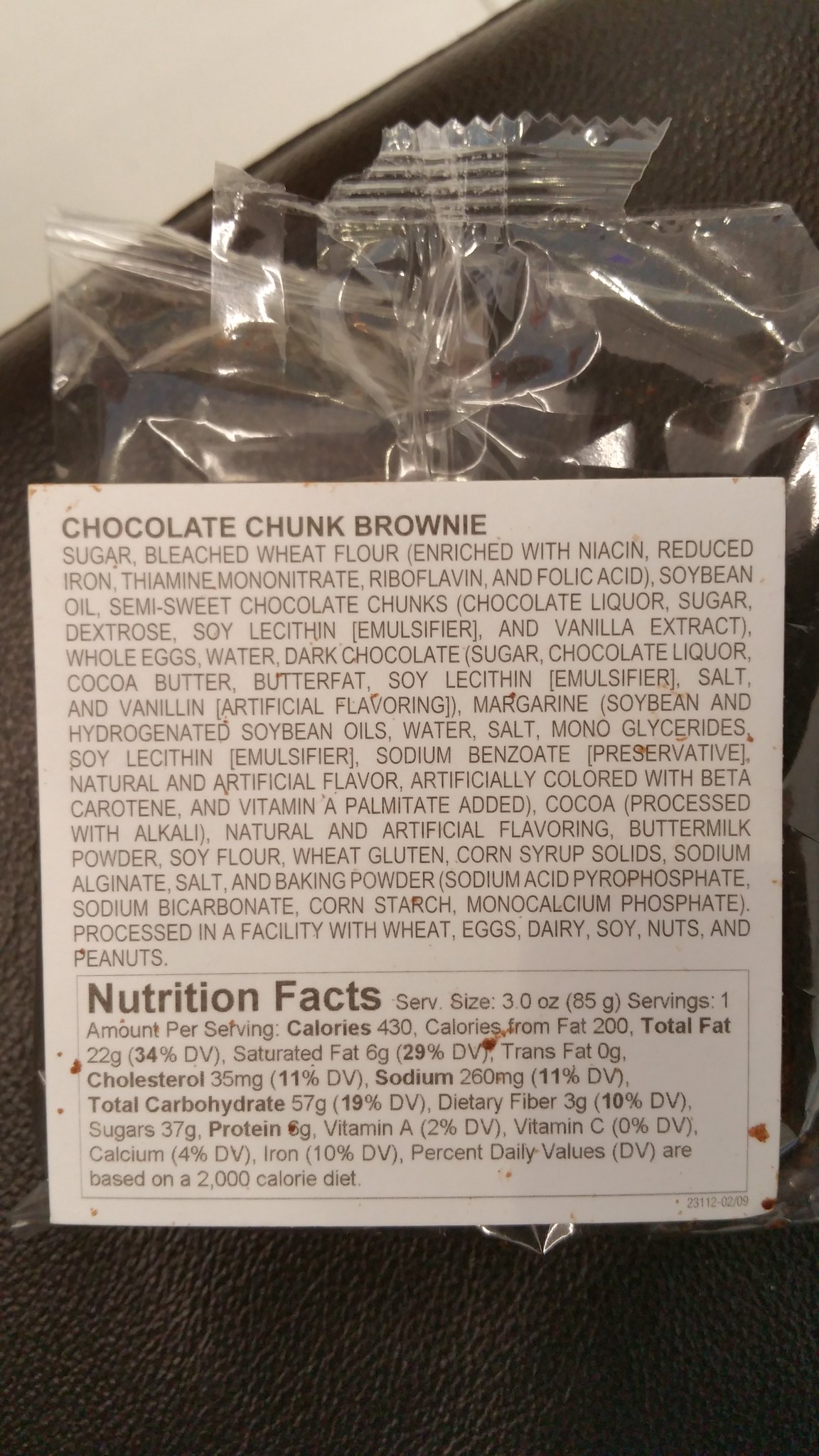The image shows the back of a package for a Chocolate Chunk Brownie, encased in a clear plastic wrapper with a slightly torn top. The label, which is square and prominently displayed, reveals a comprehensive list of ingredients and nutrition facts. The top part of the label lists ingredients such as sugar, bleached wheat flour enriched with iron and folic acid, semi-sweet chocolate chunks, salt, baking powder (sodium acid), and cornstarch. It also notes that the product is processed in a facility that handles wheat, eggs, dairy, soy, nuts, and peanuts. Below, the nutrition facts are in bold black text, detailing a serving size of three ounces, with 35 milligrams of cholesterol, 22 grams of total fat, and 57 grams of total carbohydrates. The package rests on a black surface with a noticeably bumpy texture.